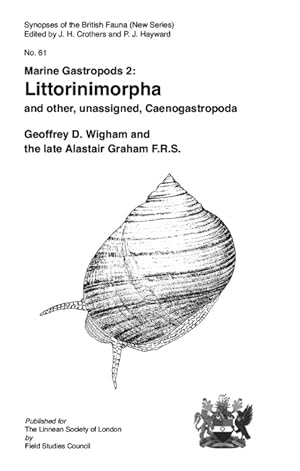This black-and-white illustration is a detailed scientific drawing of a snail, prominently featured in the center of the image. The drawing is characterized by a precise, sketch-like design typical of old scientific textbooks. In the top right corner, the text "Marine Gastropods 2" is displayed, along with a family crest featuring a crow and a lion. The illustration is part of the "Synopsis of the British Fauna New Series," as noted at the top, and is numbered 61.

The image includes a variety of scholarly details: it states that it is published by the Linnean Society of London in collaboration with the Field Studies Council. It is edited by J. H. Crothers and P. J. Hayward. Additionally, it features the text "Littorinimorpha," which is prominently bolded, followed by the phrase "and other unassigned Caenogastropoda," indicating the specific focus of the document. The authors credited are Jeffrey D. Wigham and the late Alistair Graham, F.R.S. The overall presentation suggests this image might be from a textbook or an encyclopedia focused on marine biology, particularly detailing marine gastropods.